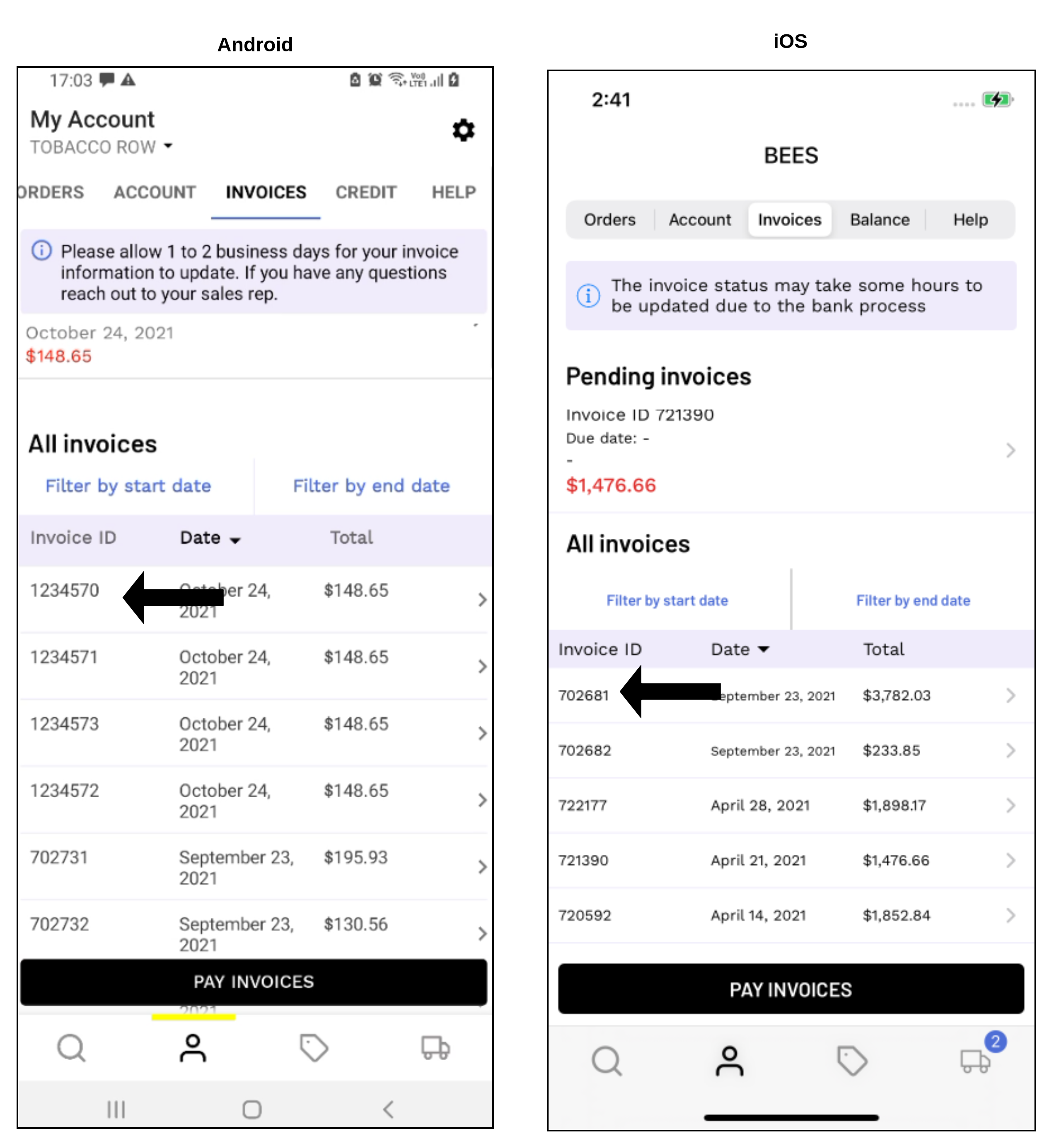### Detailed Caption:

The image displays two side-by-side screenshots from a financial application, shown on an Android phone (left) and an iOS phone (right). The app appears to be designed for managing the accounting and finances of a small business, specifically focusing on invoice management.

### Android Phone (Left) and iOS Phone (Right):
- **Top Horizontal Menu**: Both screenshots feature a top horizontal menu with the following tabs: Orders, Account, Invoices (highlighted), Credit, and Help. The highlighted "Invoices" tab indicates that this is the currently active section of the app.
- **Invoices Section**:
  - Below the top menu, there are sub-categories related to invoices such as "All Invoices" and "Pending Invoices."
  - The screen displays various details pertinent to invoicing like Invoice ID, Date, and Total Amount.
- **Bottom Navigation Bar**: 
  - A horizontal black bar at the bottom of both screens reads "Pay Invoices" in white text, suggesting a quick action function.
  - Beneath this bar are four smaller icons:
    - A gray magnifying glass (search button) on the far left.
    - A black silhouette of a person, indicating the active tab.
    - A gray shopping tag, potentially for items or orders.
    - A gray truck, likely representing deliveries or shipments.

These thoughtfully designed elements form a user interface that is consistent across both Android and iOS systems, ensuring ease of use for users managing business finances and invoices on either platform.